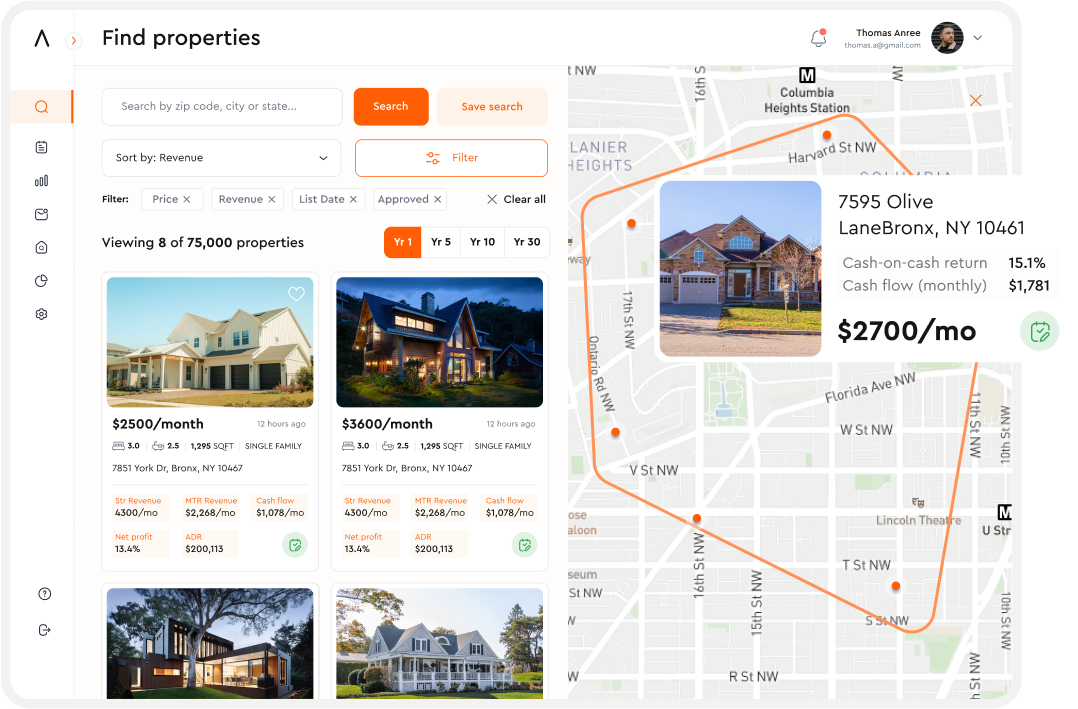The screenshot is of a property search application designed for desktop use, shown in a landscape format ideal for a computer screen rather than a mobile device. The interface features a light gray border with rounded corners, giving it a modern look. At the top of the screen, there is a header with the text "Find Properties" in bold black font.

A vertical toolbar is positioned along the left side, with a prominent search icon enclosed in an orange box and a dark orange vertical line, indicating that it is currently selected. To the right of this toolbar is a wide column dedicated to search and filtering options. Users can search for properties by zip code, city, or state using a prominent orange search button.

Filter options in this column include "Price," "Revenue," "List Date," and "Approved Viewing." There is a highlighted button labeled "Year One," which is also in orange. The current view shows the user sorting properties by revenue, with a total of 75,000 properties available for browsing.

On the right side of the screen, a map is displayed, featuring a five-sided polygon that marks a specific searched area. One highlighted property within this area is listed as "7595 Olive Lane, Bronx, New York," available for $2,700 per month.